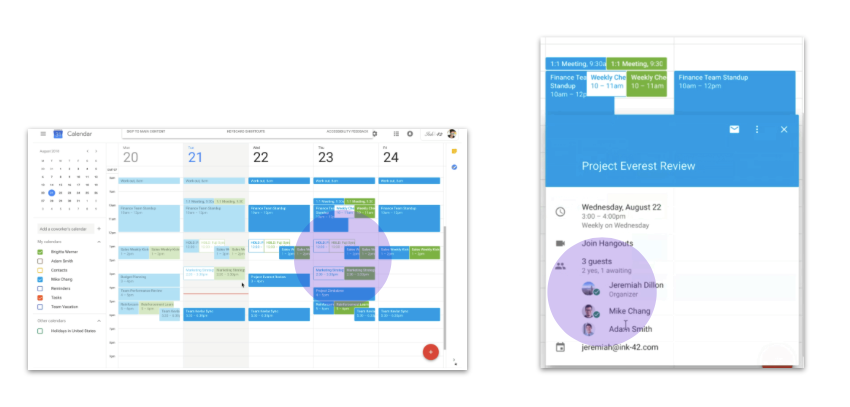The image displays a detailed, digital calendar interface. On the left side of the image, the calendar is organized by days of the week, starting with Tuesday the 21st. Each day comprises various time slots filled with different tasks and events, highlighted by blue bars and labeled rectangles.

On Wednesday, August 22nd, there are notable events such as a "Finance Team Standout" event from 10 a.m. to 12 p.m., presented in red text. This is followed by an "Envelop" marker, and a "Project Coverage Review" from 3 to 4 p.m., which occurs weekly on Wednesdays. Notification for this event indicates three guests: organizer Jeremiah L. Dillon, Mike Chang, and Adam Smith, with one guest still awaiting a response. The organizer’s email is Jeremiah at ink-42.com.

A red circle appears at the bottom right of the screen, possibly indicating an action button. A scroll bar is visible on the far right side of the calendar interface, and the border of the calendar is gray. The overall interface is meticulously organized with multiple events and tasks clearly defined in their respective time slots.